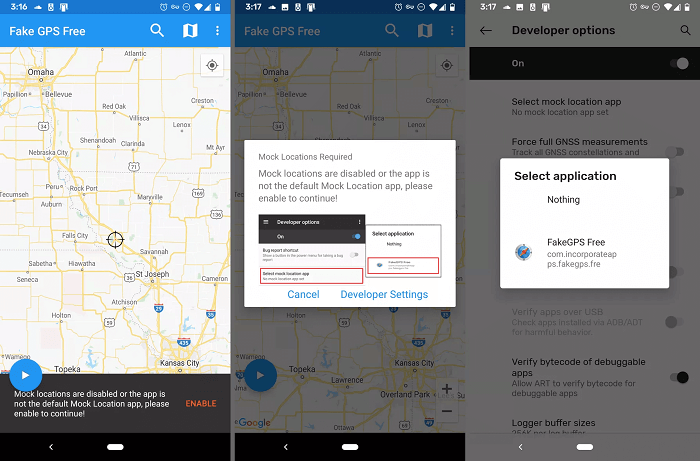The image consists of three screenshots, all of which appear to be from a mobile application rather than a desktop web page. 

1. **First Screenshot:** At the top, the heading displays the app name as "Fake GPS Free." The map visible in the screenshot resembles the interface seen in Google Maps, with a yellow-colored background. Highways and boundaries are also marked in yellow, while city names are in black. Prominent cities on this map include St. Joseph and Omaha. At the bottom of the screen, a black banner displays a message stating, "Mock locations are disabled or the app is not the default mock location app, please enable to continue."

2. **Second Screenshot:** The middle column features the same app, "Fake GPS Free," with an identical map showing yellow boundaries and black city names. A pop-up message in the center states, "Mock locations required. Mock locations are disabled or the app is not the default mock location app, please enable to continue." Additionally, it provides instructions on how to enable mock locations to proceed further.

3. **Third Screenshot:** This section provides a visual guide on how to select the correct application, "Fake GPS Free," as the default mock location app. It ensures the user knows the steps to enable the mock location setting.

Overall, the detailed screenshots aim to guide users on configuring their device settings to enable the "Fake GPS Free" application for mock locations.